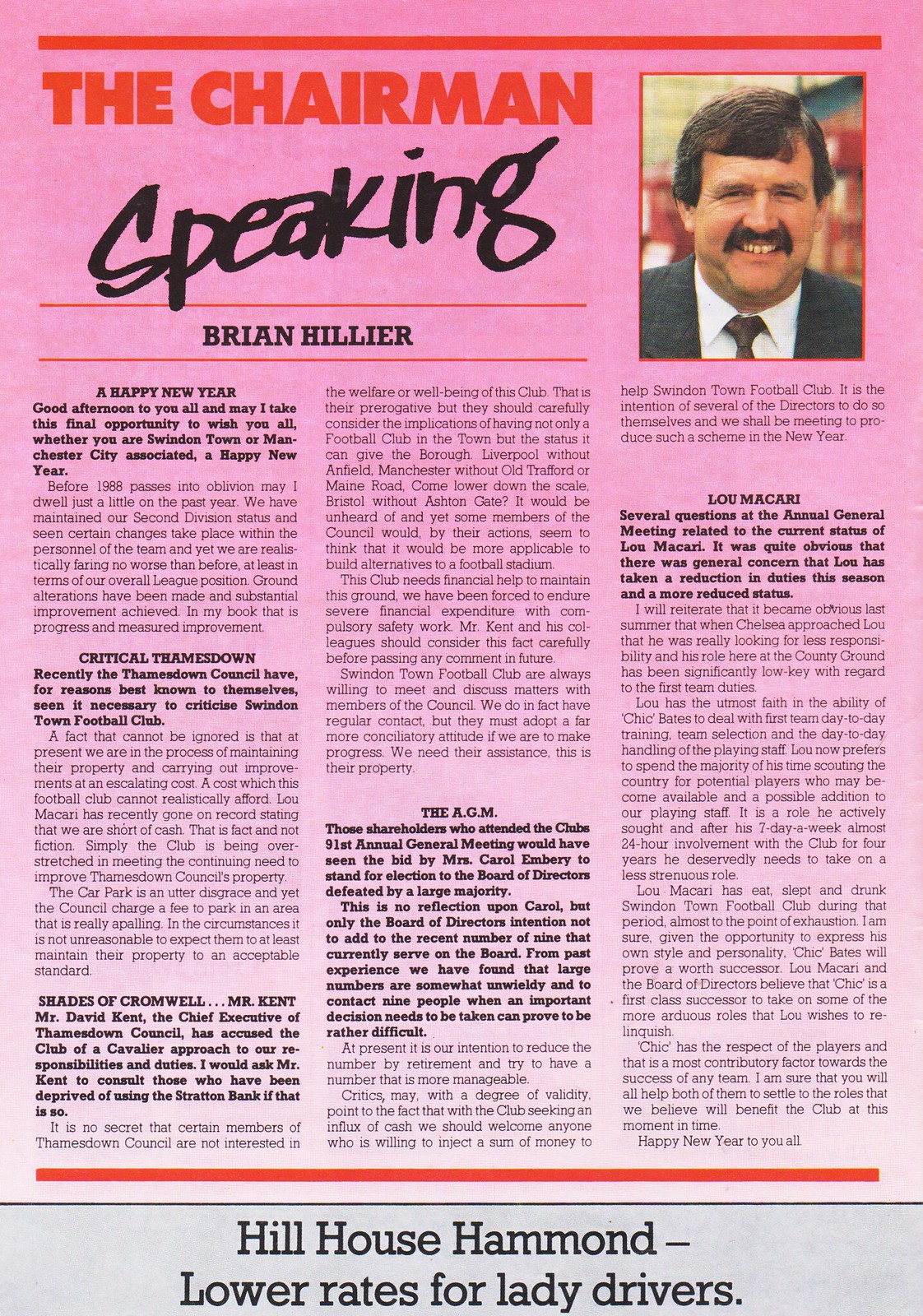The image depicts a page from an old corporate newsletter or magazine featuring a prominent article titled "The Chairman Speaking" by Brian Hillier. The page has a distinctive pink background with a gradient that transitions to a lighter pink towards the bottom. At the top of the page, a red stripe holds the bold red title "The Chairman," followed by "Speaking" in black script.

To the right of the title is a photograph of the chairman, Brian Hillier, a white man with a thick black mustache, short black hair, and dressed in a black business suit with a white collared shirt and a dark red tie. Hillier is smiling in the photo.

The article is organized in three columns, featuring bold section titles such as "Happy New Year," "Critical," "Tamesdown," "Shades of Cromwell," "The AGM," and "Lou Macari." The text under these headings engages with various topics of relevance possibly to the company's employees or stakeholders.

At the very bottom of the page, there is a gray border with an advertisement in black lettering that reads, "Hill House Hammond, lower rates for lady drivers." This ad and the article suggest the page is from a corporate publication related to Hill House Hammond.